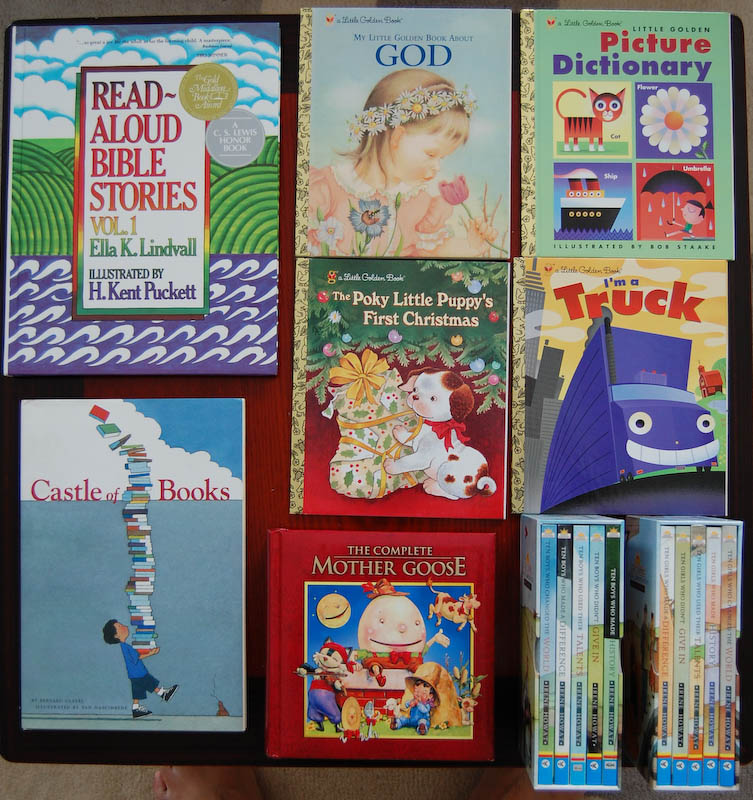This image displays a top-down view of a children's library table, showcasing an array of educational books, many with God-based themes. There are seven prominent books arranged in three columns. The top left book is "Read Aloud Bible Stories, Volume 1" by Ella K. Lindvall and illustrated by H. Kent Puckett. Below it is "Castle of Books". In the center column, the top book is "My Little Golden Book About God," followed by "The Pokey Little Puppy's First Christmas" and "The Complete Mother Goose". On the top right is "Little Golden Picture Dictionary," with "I'm a Truck" positioned below it. Additionally, there are two containers, each holding a series of five books, suggesting they belong to a set. The perspective reveals someone's bare feet at the bottom, reinforcing the relaxed, inviting nature of the children's library setting.